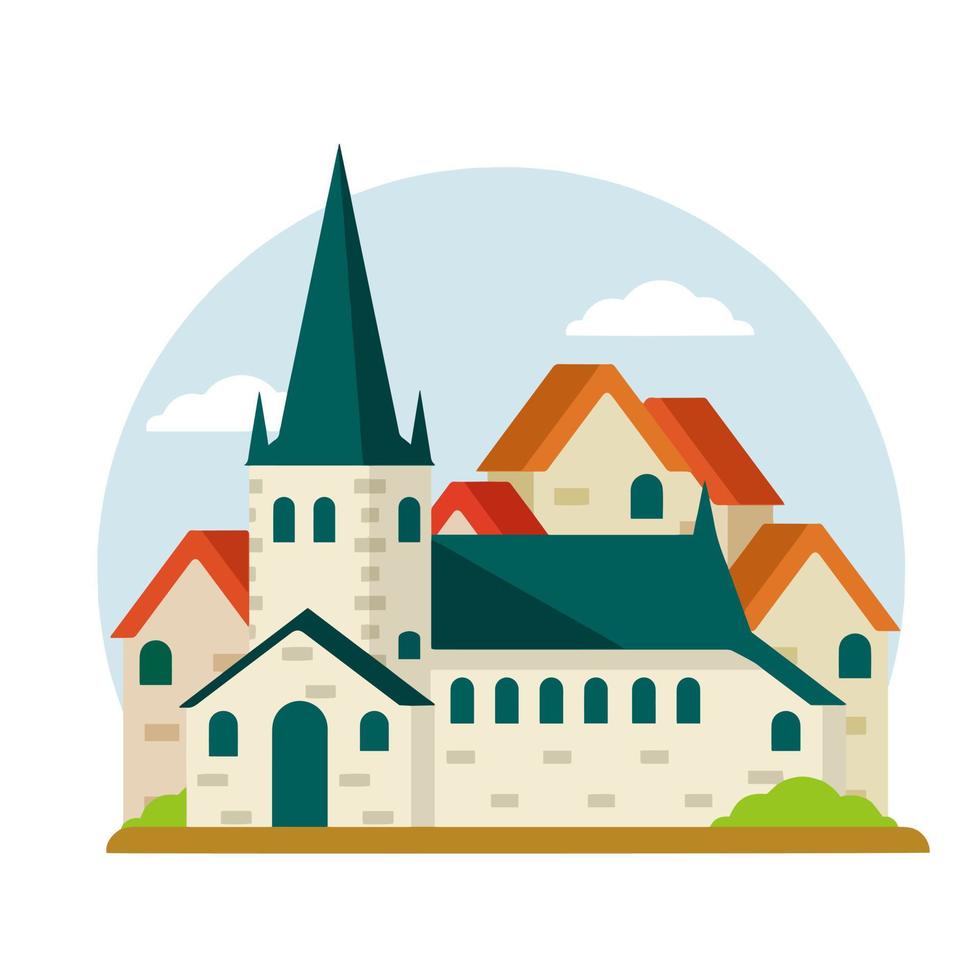This cartoon-like digital rendering depicts a picturesque village scene with a prominent castle-like building at the forefront. The central structure, which resembles a church or cathedral, features a striking green roof with a tall pointed section and a smaller adjacent roof. It boasts various long, rounded green windows, including two in the front, six along the right side, and a green door. Behind this main building, several other structures with orange and burnt-orange roofs suggest a quaint town atmosphere. Each of these buildings is adorned with green windows as well, including a cylindrical window on the leftmost structure and rounded windows on both the central and right buildings.

The background features a cyan, half-circle sky that resembles a snow globe dome, with small white clouds, one of which is partially obscured by the central building. The sky arches over the scene with a series of semicircles: a small one on each side, a medium-sized one adjoining them, and a larger central semicircle. The base of this dome-like sky image is flat, adding to the whimsical cartoon aesthetic. Additionally, the scene includes two green bushes on either side and a brown line in the front indicating a dirt path or border. The entire composition creates a charming, idyllic view of a serene village encapsulated in a semi-enclosed, snow globe-like setting.